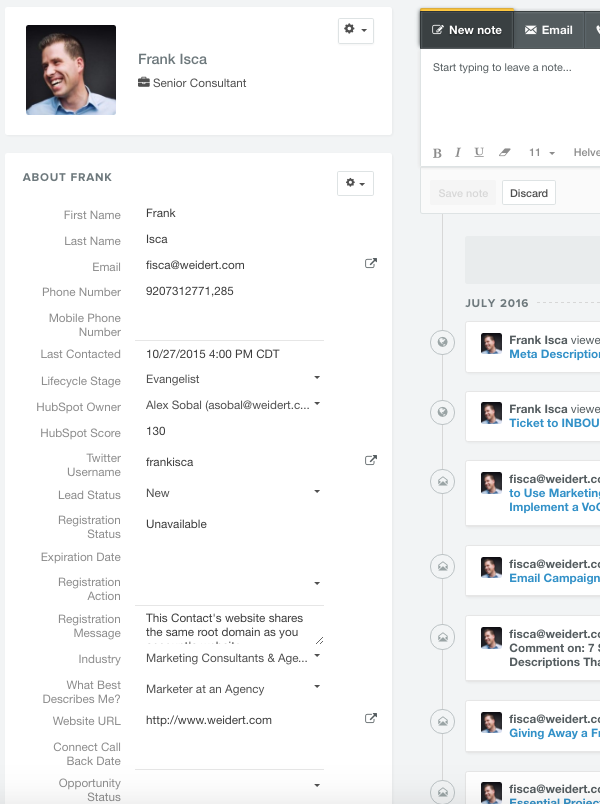The image depicts a detailed screenshot from a Customer Relationship Management (CRM) software, displaying information for Frank Isca, an ISCA Senior Consultant. The CRM entry includes comprehensive personal and professional details such as his first name (Frank), last name (Isca), email address, phone number, and mobile number. Additionally, it logs the last contact date, life cycle stage, associated Sage software, and the HubSpot owner responsible for the account. Frank's profile also includes a lead score, his Twitter username, lead status, registration status, and expiration date. The interface is set against a white background and features a small profile picture of Frank Isca, aiding in the visual identification within the CRM. The captured screenshot offers a clear view of how the CRM organizes and presents vital contact information for efficient management and follow-up.